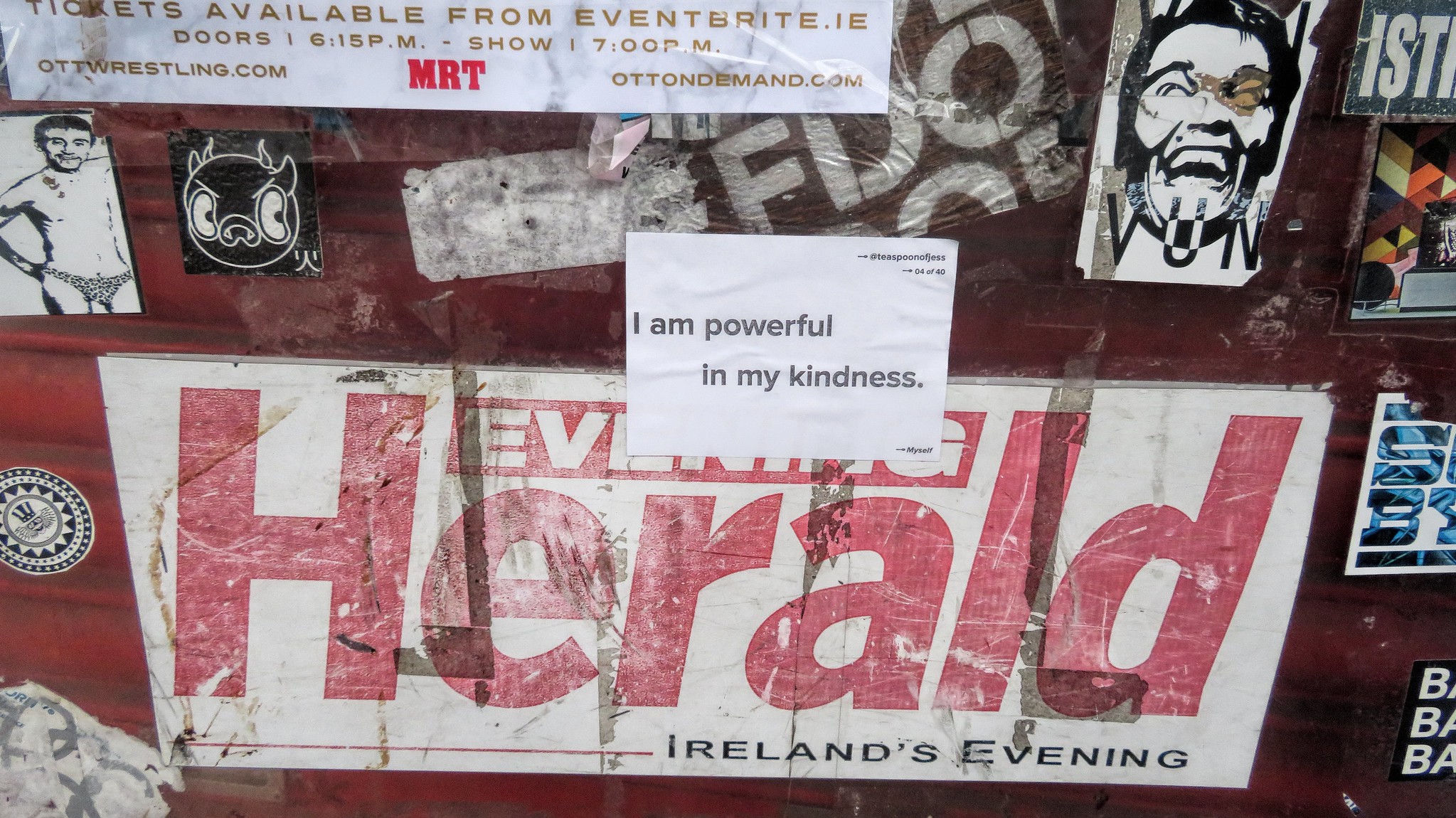The image captures a window covered with a collage of various pictures and advertisements. Dominating the scene is a well-worn white poster with red and black text that reads: "Evening Herald" in red, followed by "Ireland's Evening" in black underneath. A laminated white square with the phrase "I am powerful in my kindness" in black font partially covers the top of the poster. Nearby, a cartoonized figure resembling Arnold Schwarzenegger is depicted on a small piece of black paper. To the left, there is a sketch of a man in underwear or a bikini on a white background. Prominently displayed is also a sign indicating "tickets available from Eventbrite" in white and brown text. Additional cartoon-style stickers add to the eclectic mix, all set against a red backdrop visible through the glass, giving no clear indication of the setting behind this colorful array.